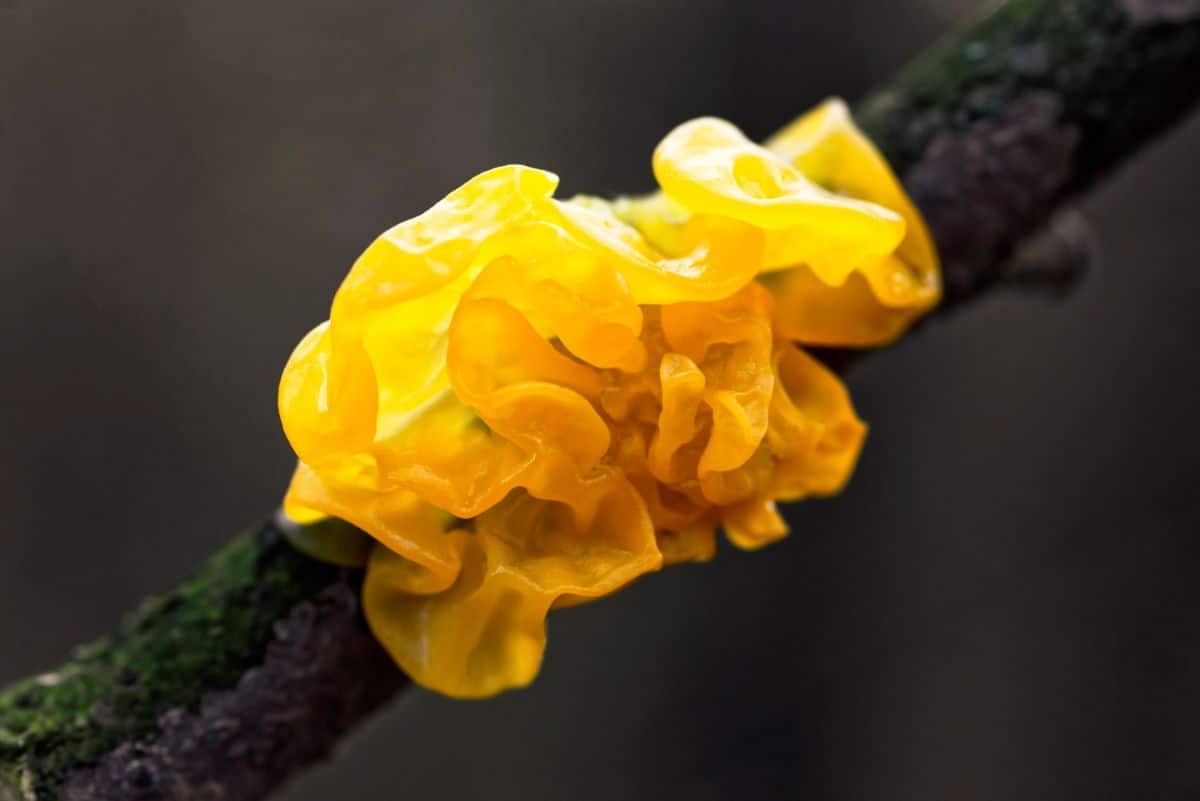The image captures a close-up of a dark tree branch, which diagonally extends from the lower left to the upper right corner. Adorning the branch is a vivid, golden-yellow fungus, identifiable as a type of jelly fungus, possibly the yellow brain, golden jelly, or witch's butter. This fungus has a folded, ruffled texture that resembles chewed-up gum and features small indents. Its translucent nature allows light to pass through, highlighting its bright yellow hue at the top and a more golden tint towards the bottom. The branch also boasts patches of very dark green moss on its upper side, while the background is a blurry gray, ensuring the focus remains on the striking yellow fungus. The overall photographic style is one of detailed realism, emphasizing the intricate textures and colors of the subject in a landscape orientation.